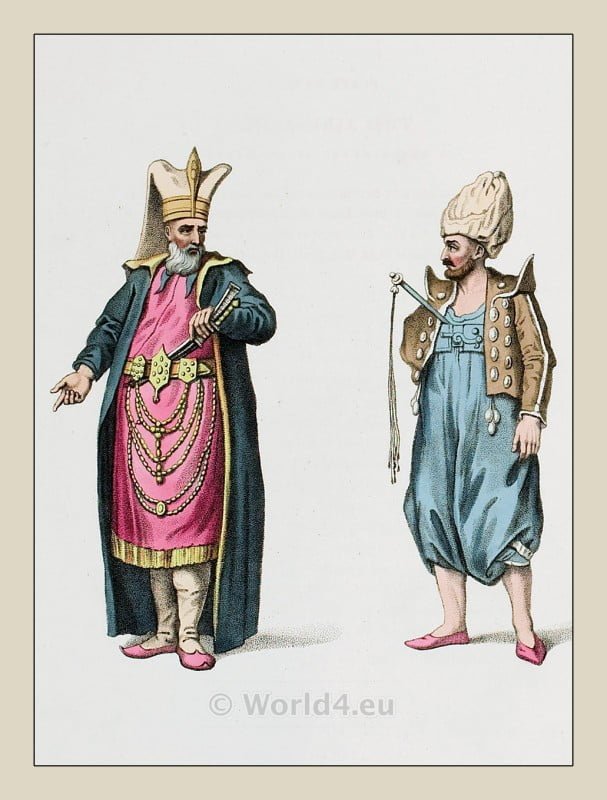This detailed illustration, presented on a soft grey background framed by a tan-ish beige border, depicts two bearded men standing side by side, dressed in elaborate historical attire. The man on the left wears an ornate outfit featuring a long pink dress with a gold belt adorned with chains and yellow fringe at the hem. Over this, he dons a blue long coat with gold-colored threading on the collar. His head is crowned with a tall, white hat resembling a banana peel, which has a gold piece emerging from it. His stockings are white, complemented by pink ballet slippers, and he holds a sword in his left hand, tucked into his waistband. His beard and mustache are gray and white. The second man, standing to the left, sports a voluminous blue romper resembling flowy pantaloons with pink ballerina slippers peeking out at the bottom. His attire includes a brown coat with prominent pointy shoulders and silver ornamentation, alongside a tall, wrinkled head covering that is beige in hue. A sword appears to protrude from his outfit, adding to the dramatic presentation. Both men exude an air of nobility with their detailed and richly colored garments, evoking a historical or fantastical setting. The image, marked at the bottom with "world4.eu," is set against a neutral-colored backdrop, enhancing the vividness of their attire.